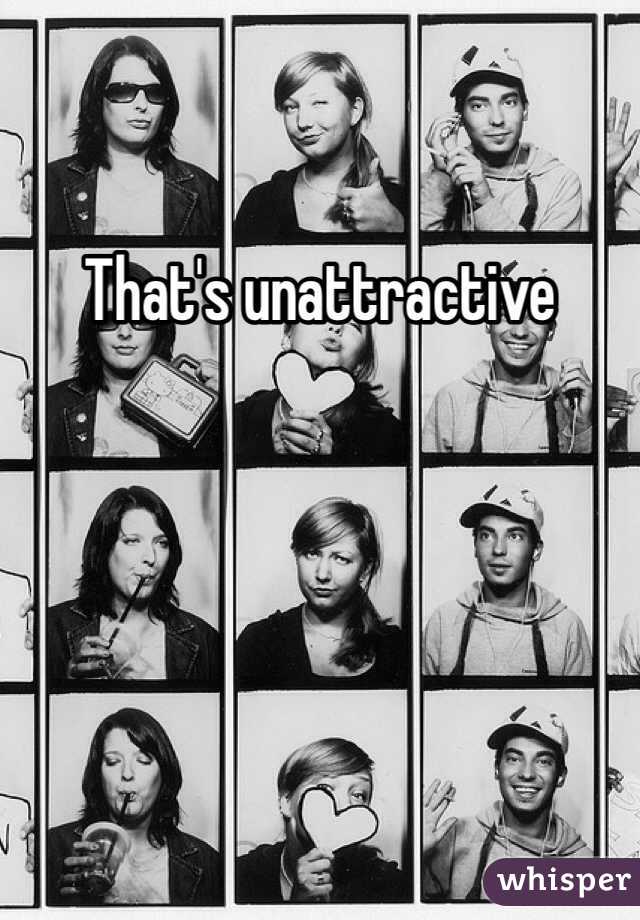This vertical rectangular image displays a grid of twelve black-and-white photographs arranged in a three-by-four pattern. The composition shows three different individuals, each captured in four sequentially unique poses within their respective vertical columns. Each person is featured with various objects and expressions, highlighting different activities. 

The left column showcases a woman with short black hair, appearing with a lunchbox in one picture and drinking from a plastic cup with a straw in two of the others. The middle column features a woman with longer hair, prominently holding a heart, suggestive of a Valentine’s theme. The right column focuses on a man, seemingly attempting to look nice while playing with his headphones across all four images. 

Across the top of the images, bold text reads, “That’s unattractive,” while additional text in the bottom right corner, set against a purple background, simply states, “Whisper.” The image series seems to be cropped, suggesting there are more photographs originally that are not visible in this view.